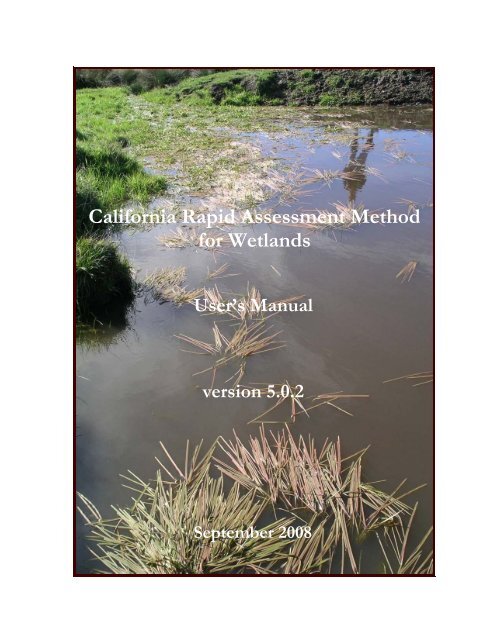The image shows a serene natural scene. In the upper right-hand corner, vibrant green grass is prominently visible. As the view extends across the frame, the grass appears to be either growing in or lying gently on a body of water. The water, though somewhat ambiguous in its form—possibly a pond—has a slightly brownish hue but remains transparent enough to reveal green plant life thriving at the bottom. Twigs can be seen interspersed throughout the scene. Superimposed on this nature image, white text reads: "California Rapid Assessment Method for Wetlands. Use this manual. Version 5.0.2, September 2008."